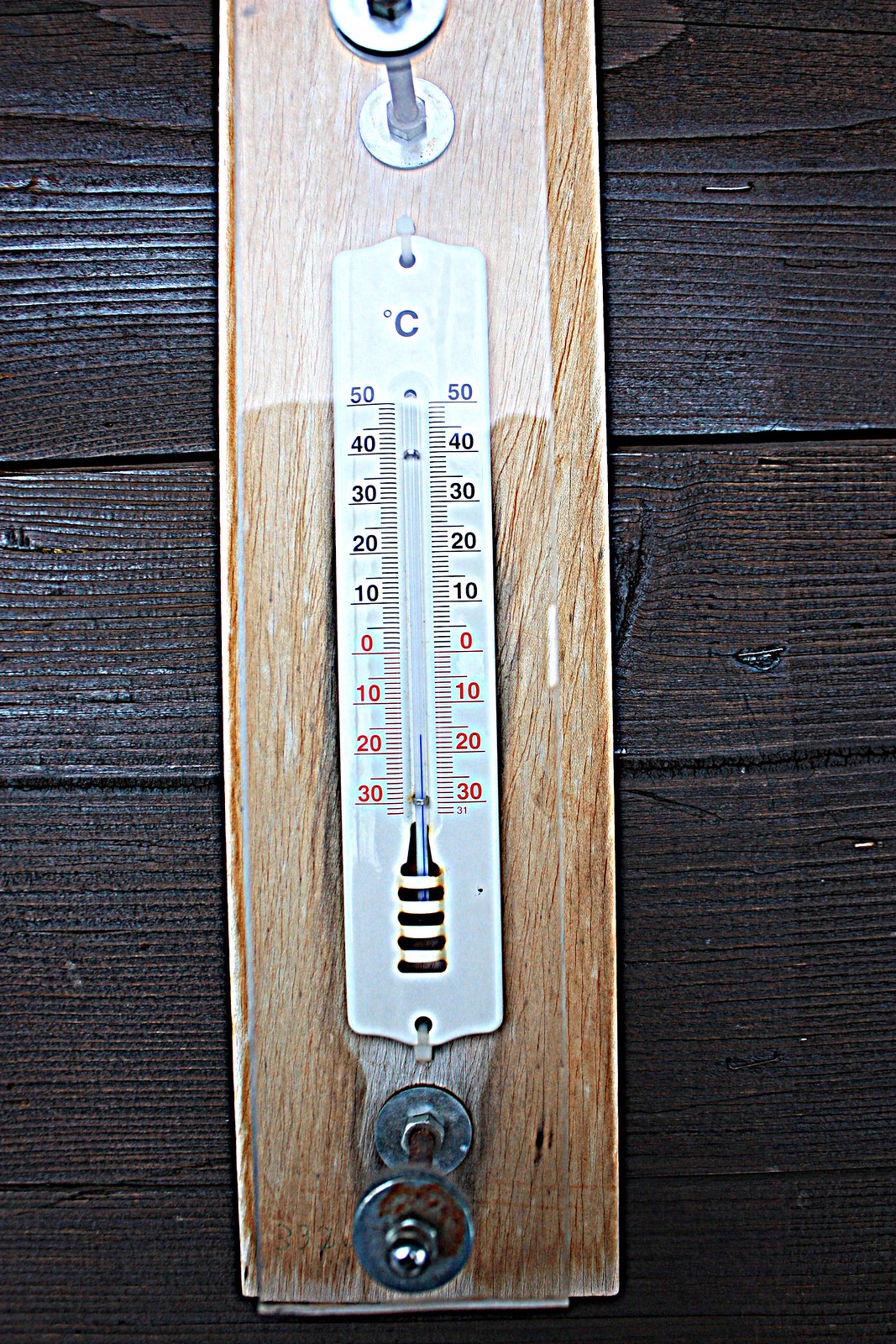This outdoor photograph features a rustic piece of dark wood-based architecture, possibly part of a building or fence, characterized by a rich, dark varnish that enhances its natural grain and texture. Affixed to the wood is a vintage-looking metal thermometer, ingeniously crafted from what appears to be an old tongue-and-groove plank. Small nails secure the thermometer to the wood, and an additional layer of protection is provided by a piece of plexiglass, held firmly in place by large bolts at both the top and bottom.

The thermometer itself is white, displaying temperature readings in degrees Celsius. The scale ranges from 50°C down to -30°C, with markings in black until it reaches 0°C, at which point the numbers turn red, likely to indicate freezing temperatures. Below the temperature scale, there is a striking yellow and black striped area, adding a visual emphasis to the critical temperature zone. The combination of materials and colors, along with the ingenuity of the design, create a visually captivating and functional outdoor piece.